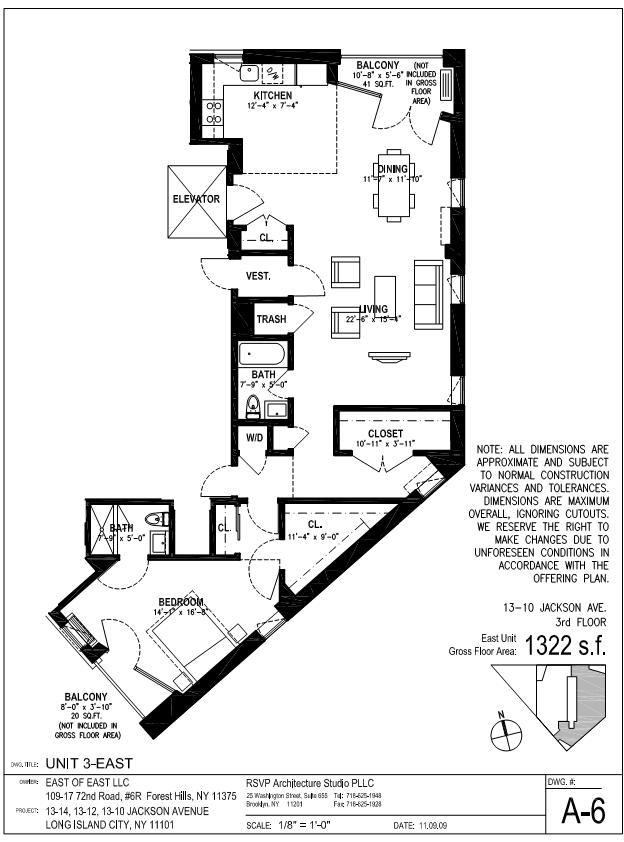Detailed Floor Plan Description for a Residential Unit

This image is a detailed floor plan for Unit 3 East, located at 13-10 Jackson Avenue, Forest Hills, New York, designed for a project in Long Island City by RSVP Architecture Studio P, LLC, designated as Drawing A-6. The unit has a gross floor area of 1,322 square feet and is rectangular at the top, tapering at an angle approximately two-thirds down, creating a leftward extension of the lower rooms.

The top section of the floor plan features an integrated kitchen, dining room, and living room, forming one expansive, open-concept area. The kitchen is positioned on the uppermost side of this section and includes modern amenities. Adjacent to the kitchen is an elevator with a swing-out door that leads directly into the unit, accompanied by a nearby closet for additional storage. A vestibule is marked in proximity, containing a trash chute for convenient waste disposal.

A balcony, slanting to the side, extends from the dining room, offering outdoor space accessible from the main living area. Within this spacious layout is a full bathroom equipped with a tub, toilet, and sink, positioned towards the central living area.

Moving to the angled extension of the floor plan, this area hosts a secondary entrance leading into a hallway lined with functional amenities. Upon entry, there is a closet, followed by a washer-dryer unit with two additional closets providing ample storage. This hallway leads to a bedroom featuring its own private balcony, enhancing the living space with outdoor accessibility.

Adjacent to the bedroom is a second bathroom that includes a shower, toilet, and sink. The entire layout efficiently maximizes living space while maintaining privacy and accessibility in key areas.

A note on the side of the plan mentions that all dimensions are approximate and subject to typical construction variances and tolerances. The dimensions provided are the maximum overall, disregarding cutouts. The right to make changes due to unforeseen conditions is reserved, in accordance with the offering plan.

Each room and area within the floor plan includes precise dimensions, given in feet and inches, to provide a comprehensive understanding of the unit's layout and scale.